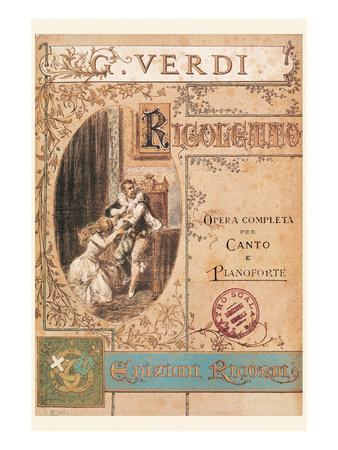The image depicts a light tan-colored poster that appears to be the cover for a play or opera. At the top, the name "G. Verdi" is prominently displayed in white lettering. Below this title, there is an illustration or painting of an emotional scene: a woman with long, orange-colored hair wearing a long dress is on her knees, seemingly begging a man who is seated, or perhaps rising, from a brown throne. The woman appears to be crying or upset. Surrounding this illustration, the poster includes a decorative vine-like border.

To the right of the image, text in Italian reads "opera completa per canto e pianoforte," suggesting that this is a complete opera score for voice and piano. There is also a notable red circular seal stamped on the lower right side of the poster, adding a touch of authenticity and formality. Additional elements include intricate, twirly floral designs on the left side and some hard-to-read text at the bottom, possibly in a blue and greenish color scheme with gold lettering.